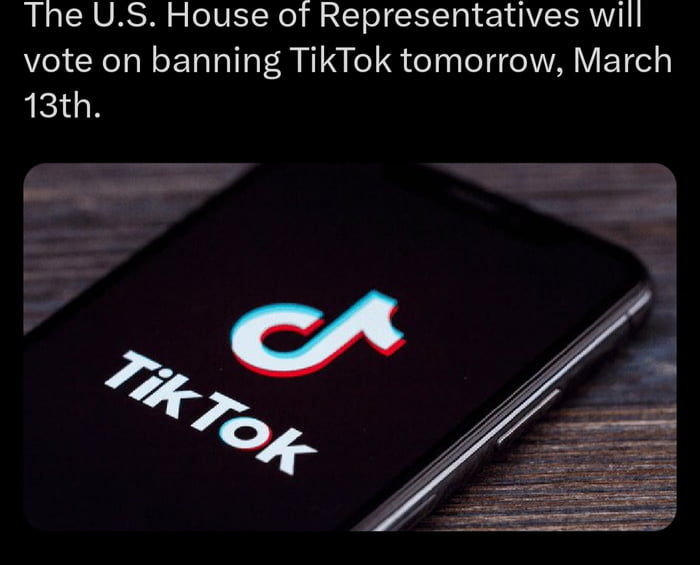The image depicts a significant announcement regarding the U.S. House of Representatives scheduled vote on banning TikTok on March 13th. The background is entirely black, providing a stark contrast to the white text at the top that reads: "The U.S. House of Representatives will vote on banning TikTok tomorrow, March 13th." 

At the center of the image is a close-up photo of a smartphone resting on a wooden desk. The phone screen prominently displays the TikTok app's logo, which is characterized by a stylized musical note resembling a combination of the 'T' and 'K' letters in the name TikTok, often compared to the Beats by Dre logo. 

The entire scene is minimalistic, focusing primarily on the text and the phone. The font used for the text is standard and easily readable. The image suggests that the announcement might be part of a Twitter post, although this is speculated. The phone's side buttons are visible, indicating a typical smartphone design. This straightforward composition underscores the gravity of the upcoming legislative decision.